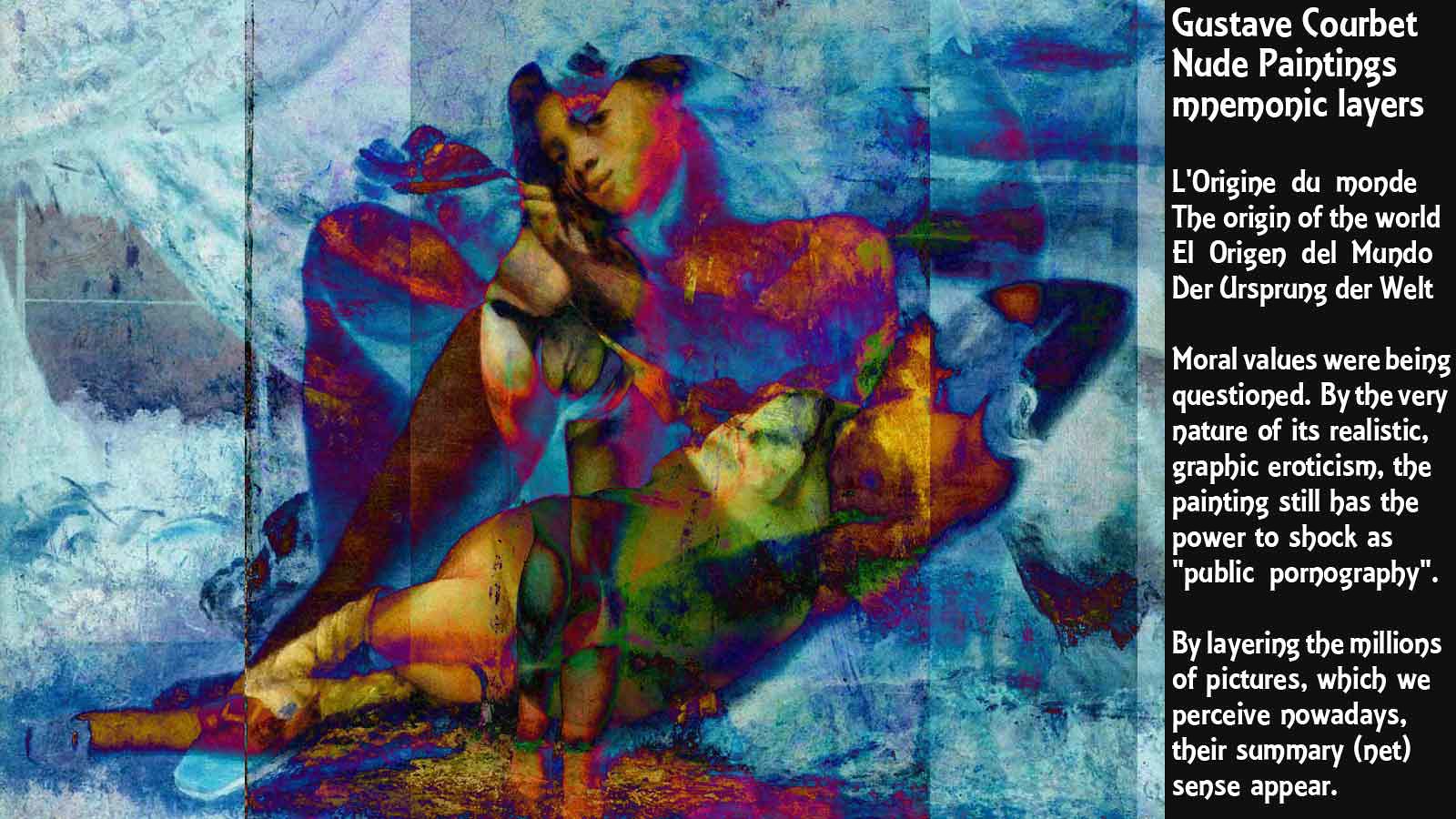This horizontally aligned rectangular image depicts a richly layered artwork, blending a swirling white and blue background reminiscent of glacial or oceanic hues. In the upper middle portion, the distinct face of a woman emerges, her body a vibrant swirl of purple, blue, and orange tones, contrasted by another, less discernible figure positioned diagonally. The background features accents of black, adding to its grainy, almost psychedelic texture punctuated by a spectrum of colors including yellow and green. To the right, a vertical rectangular section with a black background contains white text: "Gustave Courbet nude paintings, mnemonic layers." Below that, a multilingual excerpt reads: "Le origine du monde, the origin of the world, el origen del mundo, der ursprung der Welt." A final paragraph discusses the provocative nature of Courbet's work, noting its challenge to moral values through realistic eroticism that continues to shock as public pornography, and mentions the layering of myriad modern images to create a summative sense.